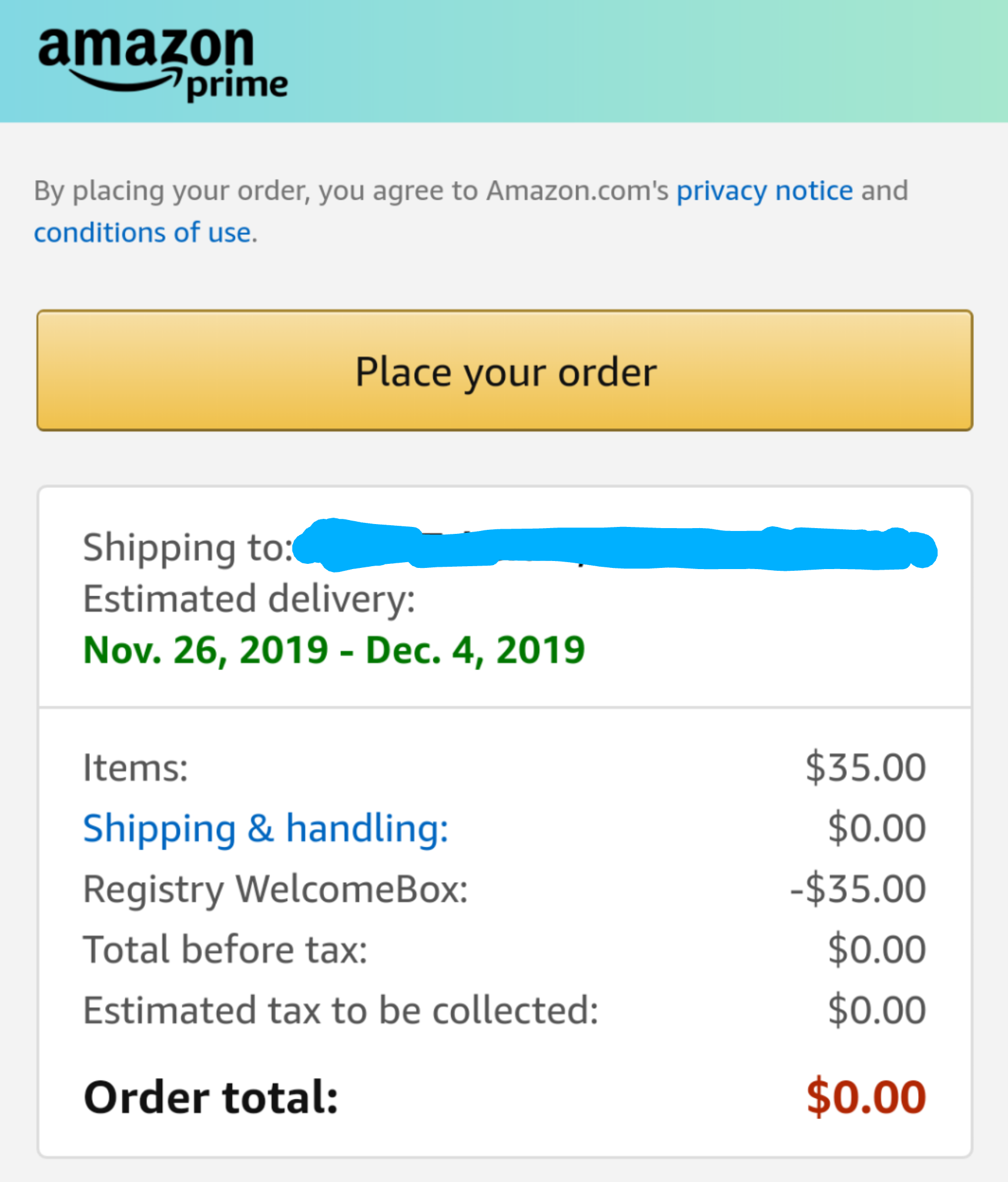This is a detailed screenshot of an Amazon order confirmation page. At the top, a lime green banner displays the Amazon Prime logo. Just below this, there's a statement on a gray background that reads, "By placing your order, you agree to Amazon.com's Privacy Notice and Conditions of Use." Centrally positioned on the page is an orange "Place Your Order" button. 

Beneath this button, a white box labeled "Shipping To" appears, with the shipping details obscured by a blue marker. The estimated delivery date is provided in green text, indicating a range from November 26th, 2019, to December 4th, 2019.

The itemized list shows:
- Items: $35
- Shipping and handling: $0
- Delivery welcome box: -$35

Consequently, the total before tax is $0, with an estimated tax of $0, making the order total $0.